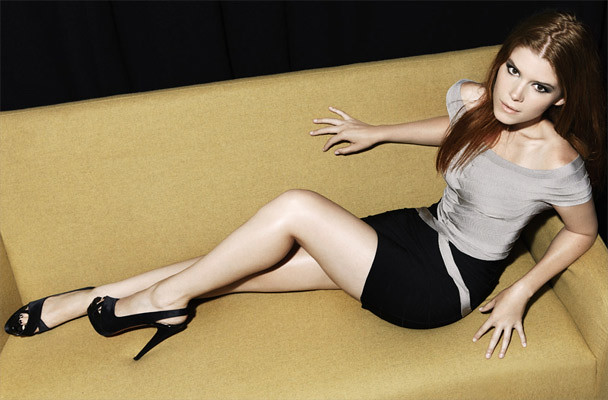In this image, we see a woman laying on a golden yellow loveseat, which occupies the entire horizontal space from left to right. The background is a solid black, enhancing the focused and intimate setting that appears to be an indoor environment with low lighting. The woman has long, reddish-brown hair and is looking directly into the camera, exuding a confident presence. She is wearing a silver shirt that exposes her collarbones, paired with a black skirt adorned with a silver line, which adds a touch of elegance to her outfit. Her black high heels, which appear to be at least five inches tall, accentuate her long legs. She has white-painted nails and brown eyes, adding to her striking appearance. The arrangement and coloration of the image emphasize her as the central figure against the contrasting dark background.